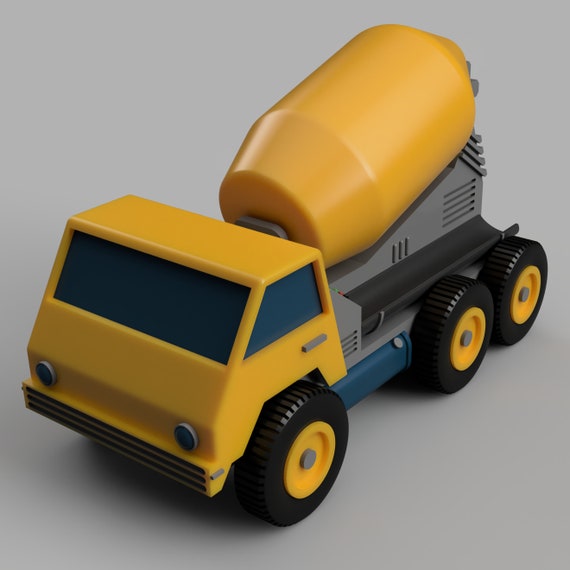The image features a close-up, indoor photograph of a toy cement truck placed in the center of a light gray background. This toy truck is depicted in a three-quarter view, highlighting its simplistic detailing. The cab and cement mixer cylinder are both yellow, with a gray body supporting the mixer. Attached below the mixing drum is a darker gray trough. The truck is equipped with six black tires featuring yellow hubcaps and includes two axles at the rear. The cab's windows and windshield are dark navy blue, and it has two gray headlights along with a black bumper. Additionally, a darkish green fuel tank is visible. The toy truck, made of smooth plastic, showcases a combination of vibrant and muted colors, providing a clear, detailed representation of a cement mixer truck that exudes simplicity and functionality.